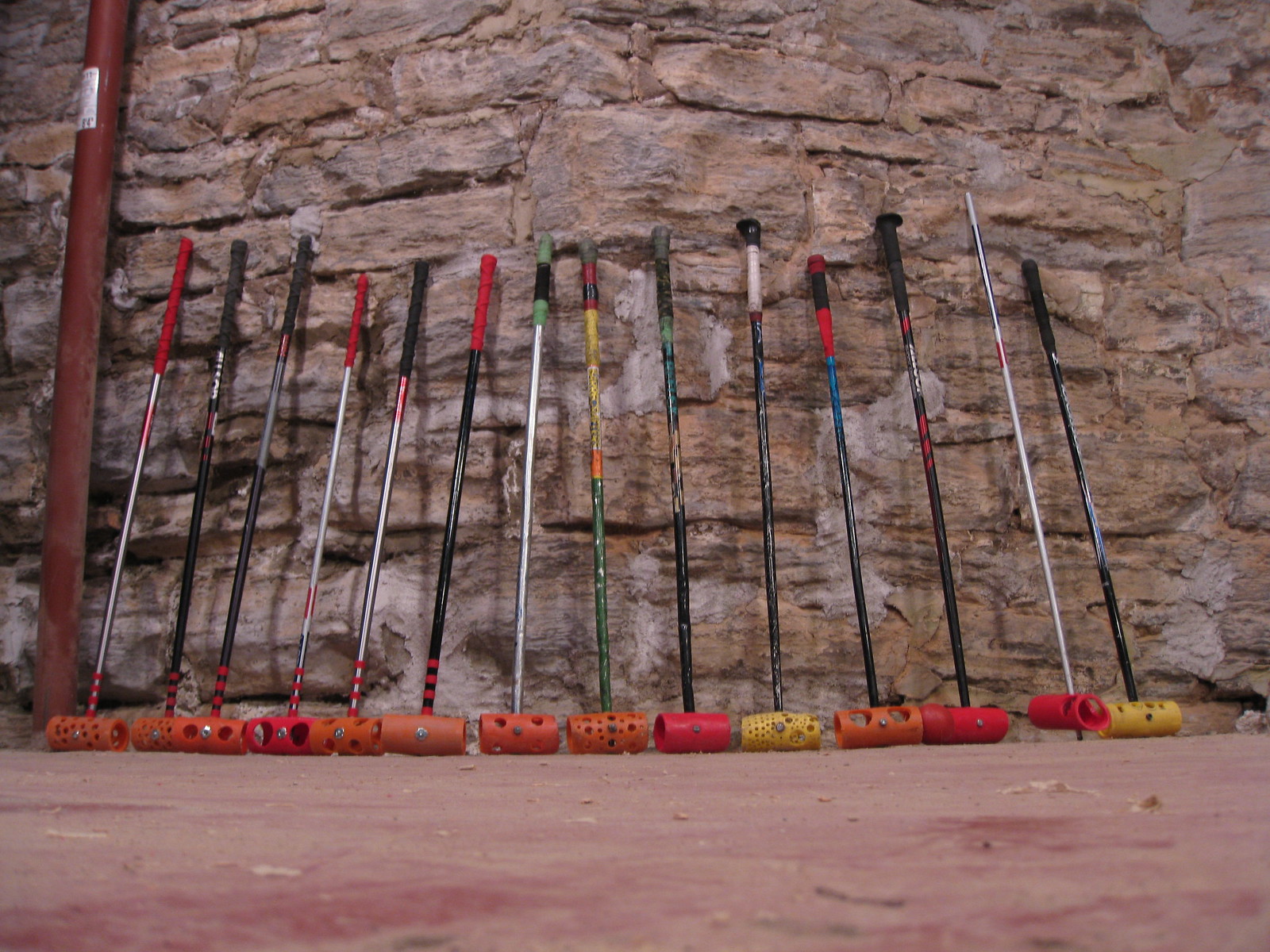The image depicts a dusty, pinkish-red sandy ground with a background of layered rock or stone that ascends upward. On the left side of the image, there's a large, burgundy pole adorned with a silver metal plaque. Along the rock wall, there are 12 cylindrical objects, possibly sports equipment resembling cricket clubs, each featuring a hollow bottom section with various holes. These cylinders are vividly colored, predominantly in shades of orange, red, and yellow, and are attached to aluminum handles. The handles vary in color, including silver, black, and one particularly unique green and yellow handle. The clubs are neatly lined up in a row, leaning against the rock wall, which shows clear cement lines between the layers, adding a rustic texture to the scene.